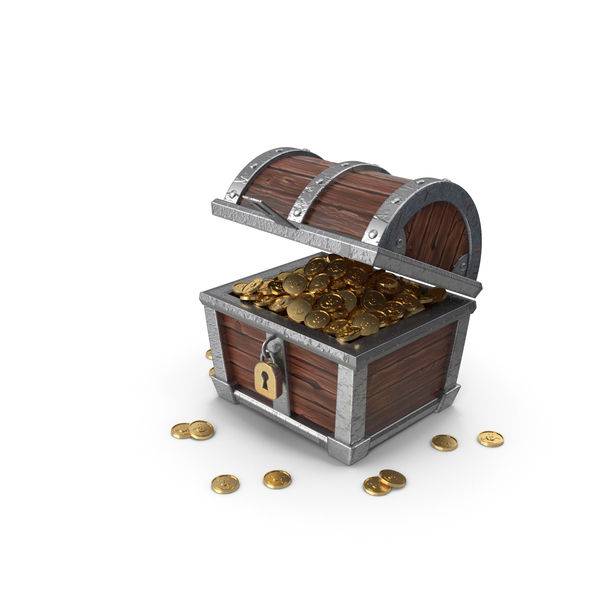This image depicts a treasure chest made of brown stained wood, adorned with three layers of silver metal backing and accented with a gold lock at its center. The chest's top, designed in a rounded semicircle form, is halfway open and seemingly resting in mid-air. Inside, the chest glimmers with numerous shiny gold coins which also spill out onto the white floor in front and to the side. The silver framework meticulously lines the borders, adding to the chest's intricate design. In total, eight gold coins are scattered outside the chest, enhancing the sense of overflowing treasure.